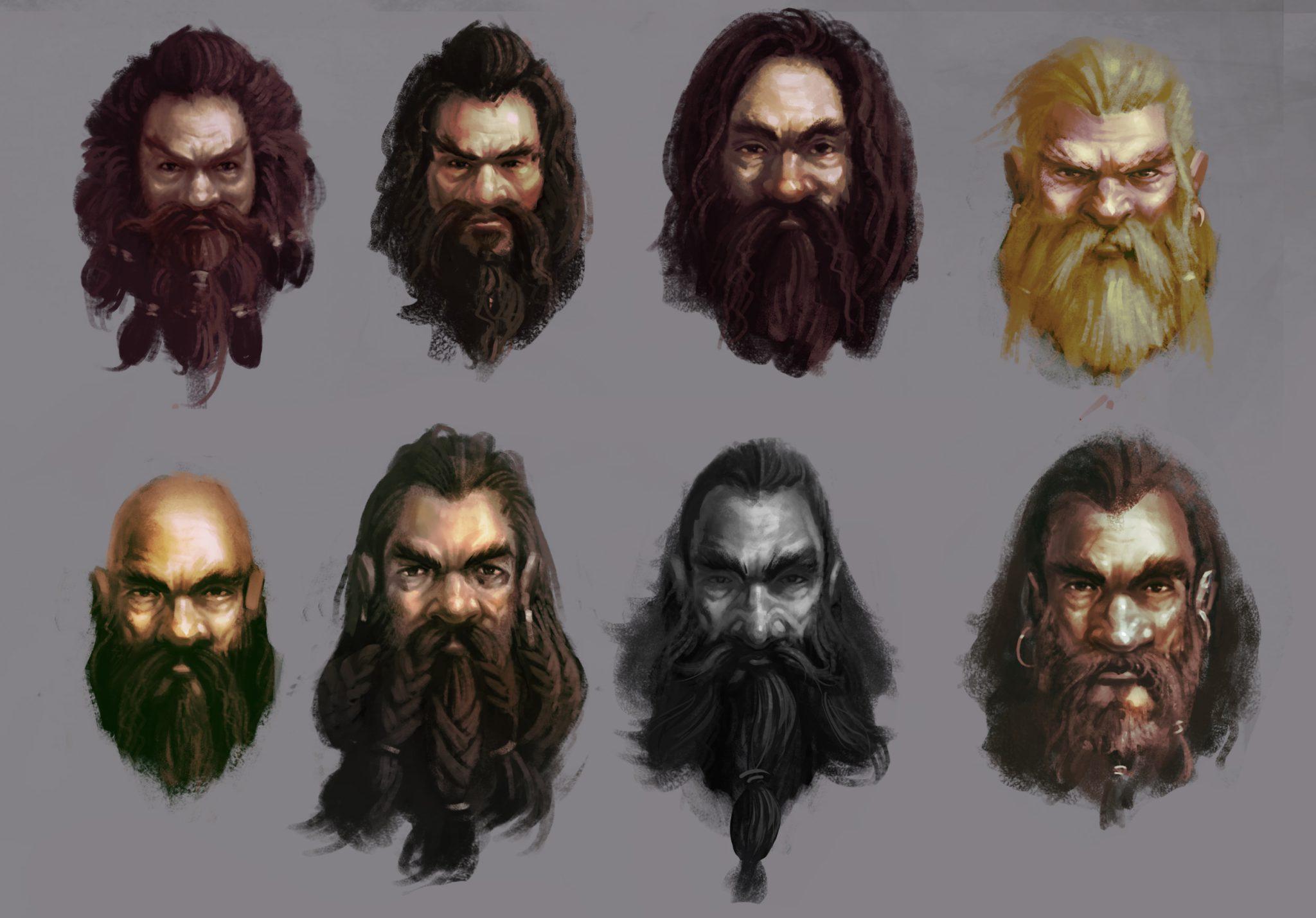This is a detailed crayon illustration featuring eight primitive or Viking-like male heads arranged in two rows of four against a light gray background. All the men display fierce, aggressive expressions, with pronounced eyebrows and sneering or menacing looks. Seven of the figures have long beards and hair, while one is bald but also sports a long beard and mustache. 

The men predominantly have brown hair, except for one who is blonde and one depicted in greyscale or black and white. Their beards vary greatly in style—some are tied into ponytails, others are braided, and a few hang loose. Each person exhibits unique details: several have earrings and ornaments in their beards, and some have braided elements.

In the top row, the first man has dark brown hair pulled back and a ponytail beard, showcasing very aggressive, pointy eyebrows. The second man, also with brown hair, looks slightly less menacing and has a small ponytail at the center of his hanging beard. The third man's appearance is shaggy and tired with dark brown hair and a loose beard, and he has a slightly grey skin tone. The fourth figure, characterized by blonde hair, has two gold earrings and two small ponytails on either side of his beard, with his hair swept back.

In the bottom row, the first face is bald with a free-flowing beard, depicting a more relaxed expression. The second man’s dark brown hair is swept back, and his beard is intricately braided into three parts; he may also be wearing earrings. The third figure in greyscale or with black hair has a thin face, shaggy eyebrows, and a long beard tied in the middle. The last man has a receding hairline, dark brown hair, and a beard divided into three ponytail sections, complemented by large hoop earrings.